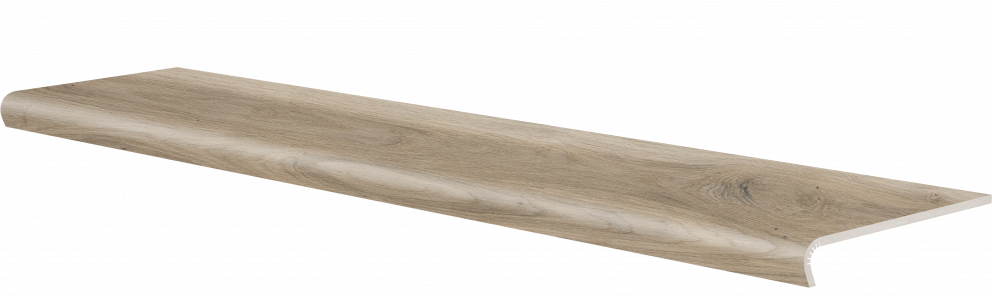This image features a meticulously crafted piece of light tan wood, set against a white background, possibly part of a piece of furniture or a countertop. The wood exhibits a smooth, professionally sanded, perhaps polished finish, highlighting its natural grain and markings. Notably, there is detailed woodgrain visible, including a knot that adds character to the material. The wood is cut in a flat shape, with its defining characteristic being a graceful curve at the front edge, which turns downwards in approximately a 100-degree curve, leaving about an 80-degree angle between the two sections of wood. This front curve serves a decorative purpose, eliminating any sharp edges and creating a sleek, professional look. The overall thickness of the wood remains consistent, maintaining a balance between function and aesthetics, making it ideal for do-it-yourself projects like a floating shelf or a countertop. The piece's straight sides and back further emphasize its potential application in various DIY or professional furniture-making contexts.